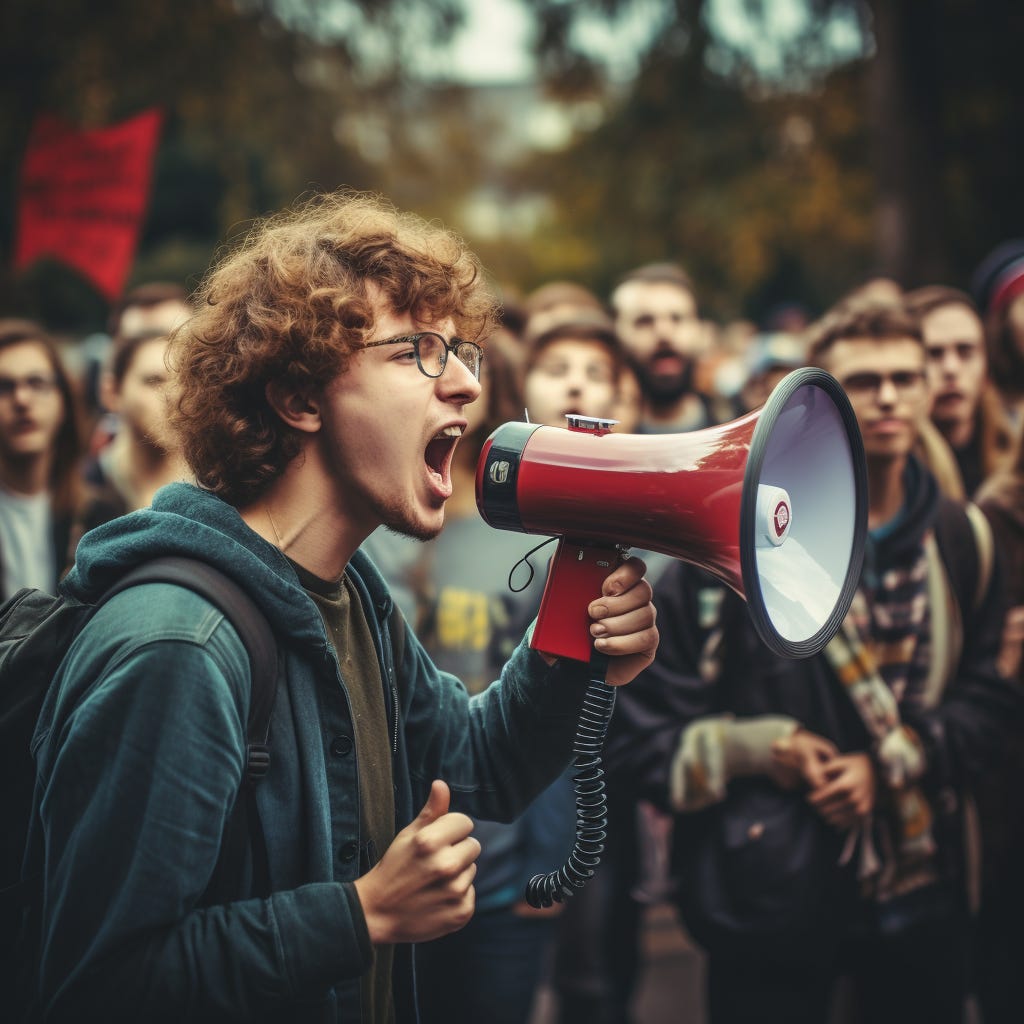In this AI-generated image, a young man with curly brown hair and black glasses is passionately yelling into a red megaphone with a black handle and a silver-black wire. He sports a blue sweatshirt over a green shirt and carries a black backpack. Despite the peculiar imperfections, like the unrealistic appearance of his hand holding the megaphone, the scene appears lifelike. Around him, numerous onlookers, dressed warmly in layered clothing, stand with varied expressions—some shocked, others intent—suggesting a politically charged or activist gathering. The background includes indistinct faces of the crowd, blurred trees, and a red sign or banner on a stick, all contributing to the vivid yet surreal atmosphere of the image.